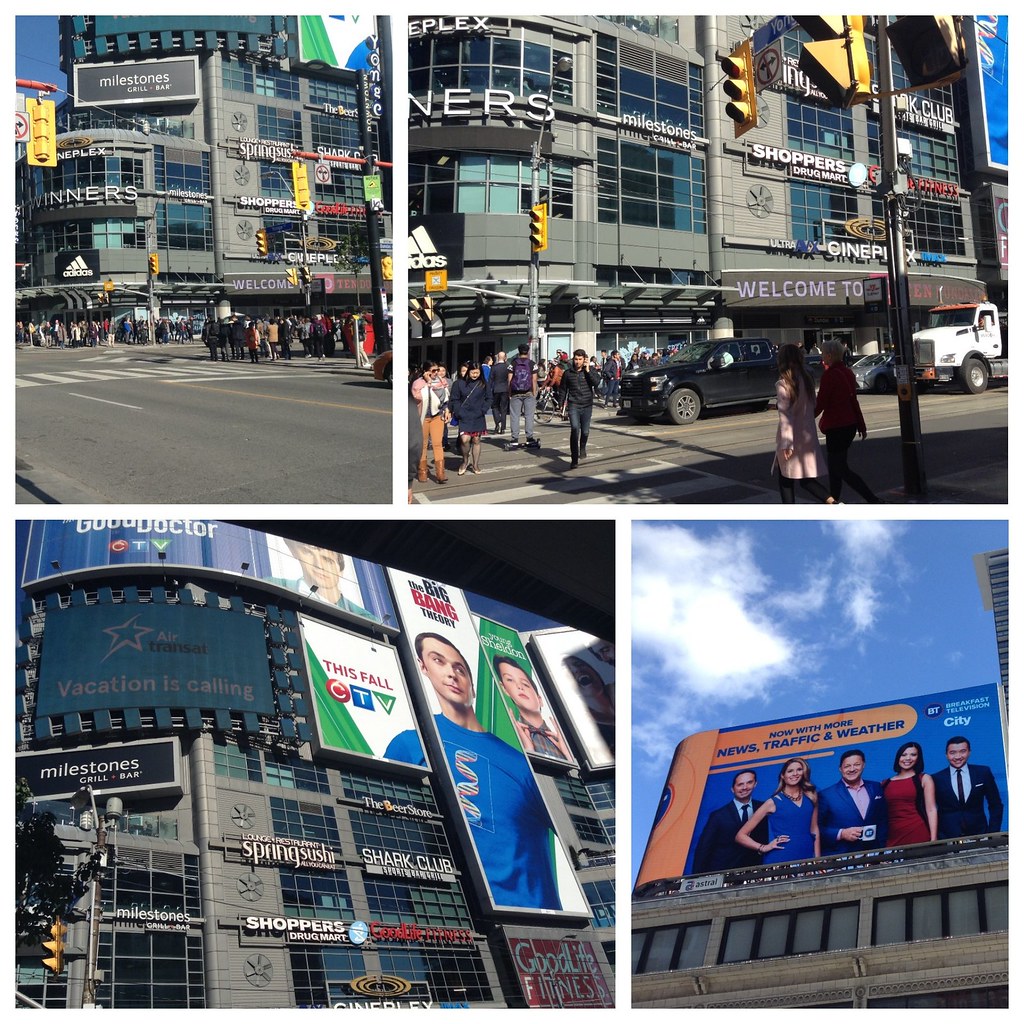The image is a collage of four full-color outdoor photographs taken during the daytime in New York City's bustling Times Square. Each picture captures a different perspective of this iconic metropolitan area. In the top left image, there are vibrant shops including Adidas, Winners, and Sharks, as well as numerous pedestrians walking down the sidewalks near some signs on a hotel. The top right image showcases a view directly across from the Adidas store, depicting a busy street scene with cars and people navigating the crosswalks amidst several traffic lights. The bottom left photograph provides an upward view from the sidewalk, highlighting more of the collection of surrounding stores. The bottom right image prominently features a large billboard for a local TV station, displaying an advertisement that reads, "Now with more news, traffic, and weather," and features five newscasters. Additional digital billboards announce popular TV shows such as "The Good Doctor," "Big Bang Theory," and "Young Sheldon," alongside another advertisement stating "Vacation is Calling, Air Transar." Numerous trucks and cars can also be seen in the images, emphasizing the area's dense traffic and vibrant urban life.